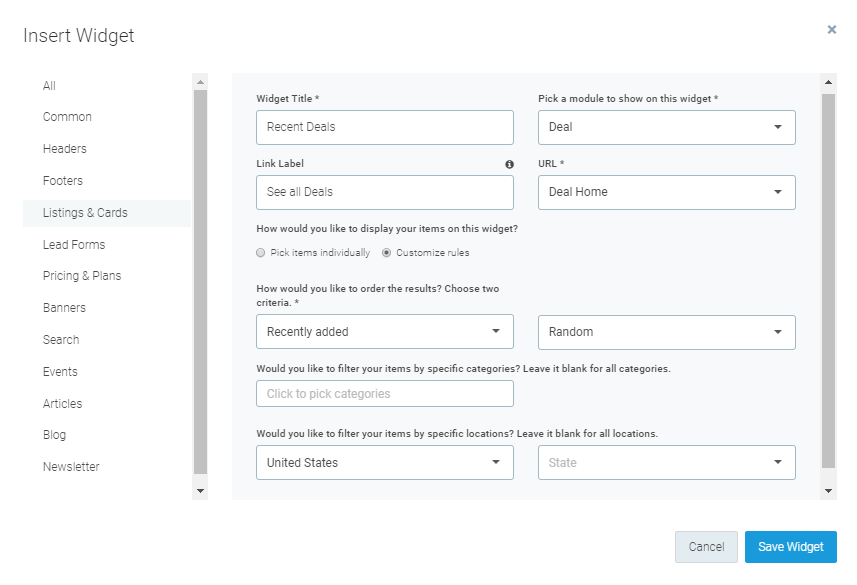A user is navigating a web page dedicated to widget creation. The interface includes a variety of options and categories in a sidebar menu to the left, prominently featuring sections like "Common Headers," "Footers," "Listings and Cards," "Lead Forms," "Pricing and Plans," "Banners," "Search," "Events," "Articles," "Blog," and "Newsletter."

The user has opted to explore the "Listings and Cards" category. Upon selection, a detailed configuration panel appears on the right side of the screen. This panel provides several editable fields and dropdown menus, allowing users to customize different aspects of the widget. Users can specify a widget title, choose a module to display, input a URL, and set other customization options.

Additionally, at the bottom of the panel, there's an option for geographic filtering, asking if users want to filter items by specific locations—left blank, this includes all locations. In this case, the user has entered "US" without specifying a state. The panel also allows users to determine the order of displayed results by choosing up to two criteria; the user has selected "recently added" and "random" as their sorting preferences.

Overall, it appears that the user is in the process of adding or configuring a widget element on their website by utilizing the provided tools and customizable options on this comprehensive web page.